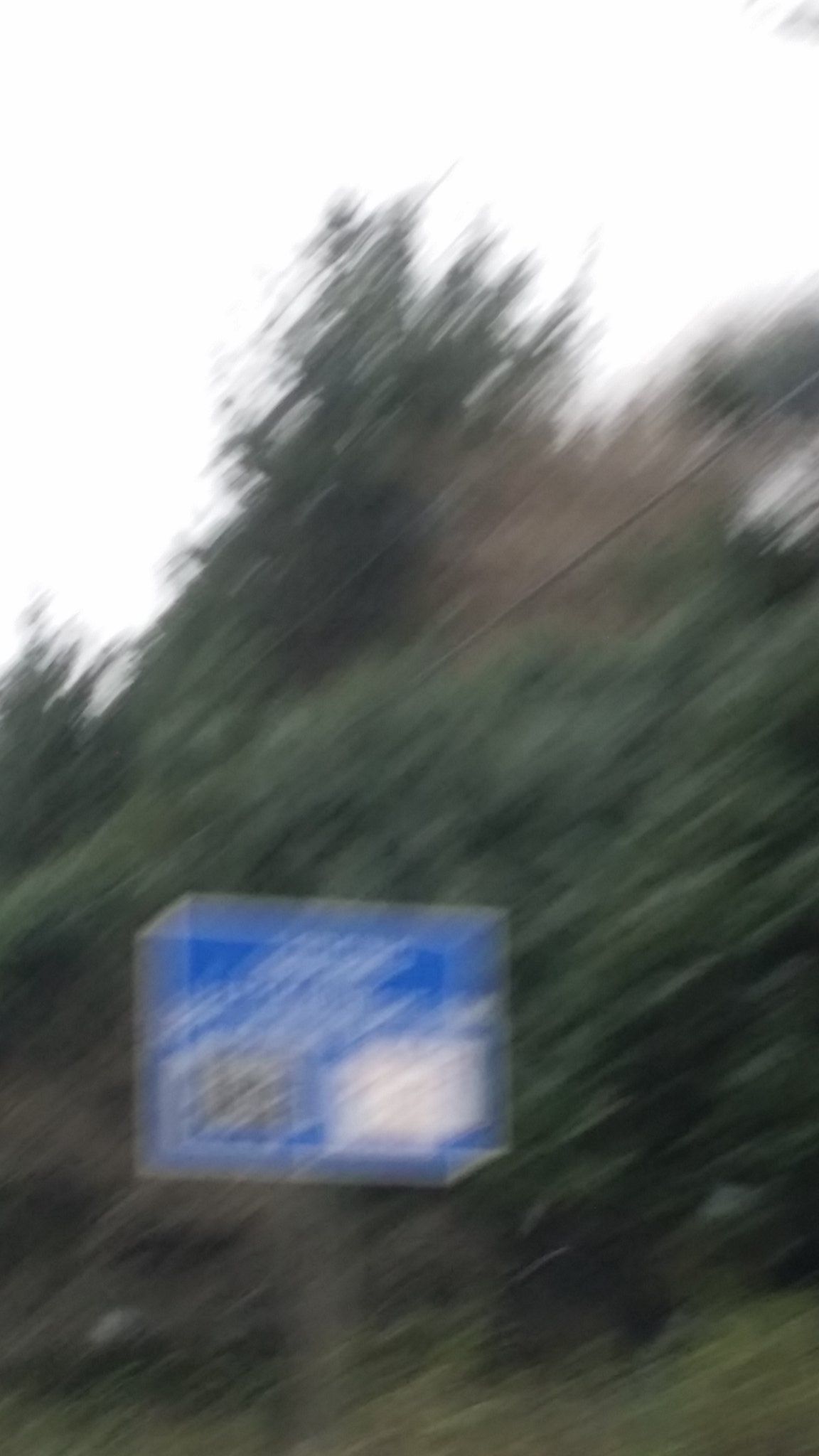This outdoor photograph captures the side of a highway. The focal point is a blue metal sign situated in front of a dense cluster of dark green trees. The sign appears to be an exit or informational sign potentially indicating the presence of amenities like a rest stop or various dining options at the next exit. Although the motion blur obscures the text, distinct features such as a black square and a white square with white lettering can be discerned. The backdrop of the scene is marked by a white, overcast sky that contrasts with the rich greenery of the trees.